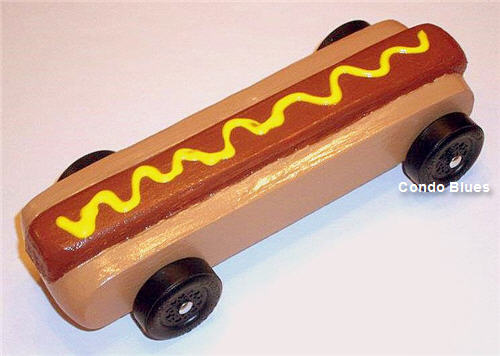This is a detailed photograph of a simplified wooden toy vehicle designed to resemble a hot dog. The car has four black wheels directly attached to a light brown wooden base that mimics a bun. At the center, a darker reddish-brown wooden piece acts as the hot dog, featuring a zigzag yellow line on top, representing mustard. The toy is angled from the bottom left to the upper right and positioned against a plain white background. Notably, the words "Condo Blues" are prominently displayed in white text below the front wheel on the upper right side. Additional details include small silver pins embedded in the hubcaps, adding to the toy’s handmade charm.